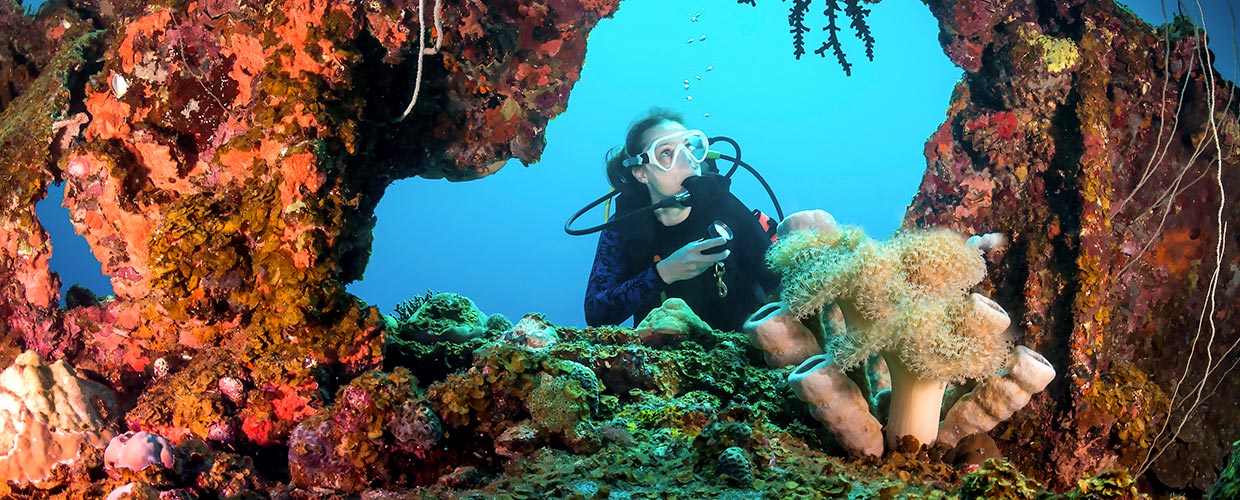This underwater photograph captures a female scuba diver exploring a coral reef. The image, taken under a coral arch, showcases a range of colors and marine life. On either side of the frame, vibrant coral formations in shades of orange, brown, and maroon-red dominate the scene. In the center, the diver, dressed in a black wetsuit and goggles, appears to be holding a flashlight in her left hand, possibly inspecting the reef. Her dark hair is visible, floating slightly in the water. Surrounding her are various types of coral, including a light cream-colored tube-like structure with fuzzy tops, and contrasting greenish patches that could be normal underwater plant life or algae. In the background, the scene is bathed in the varying shades of bright, clean blue of the ocean, with hints of greenery, possibly underwater plants or ferns, hanging down from the coral formations. The intricate details of the reef, made up of oysters, shells, and rocks, add to the rich texture and vibrant life depicted in the scene.